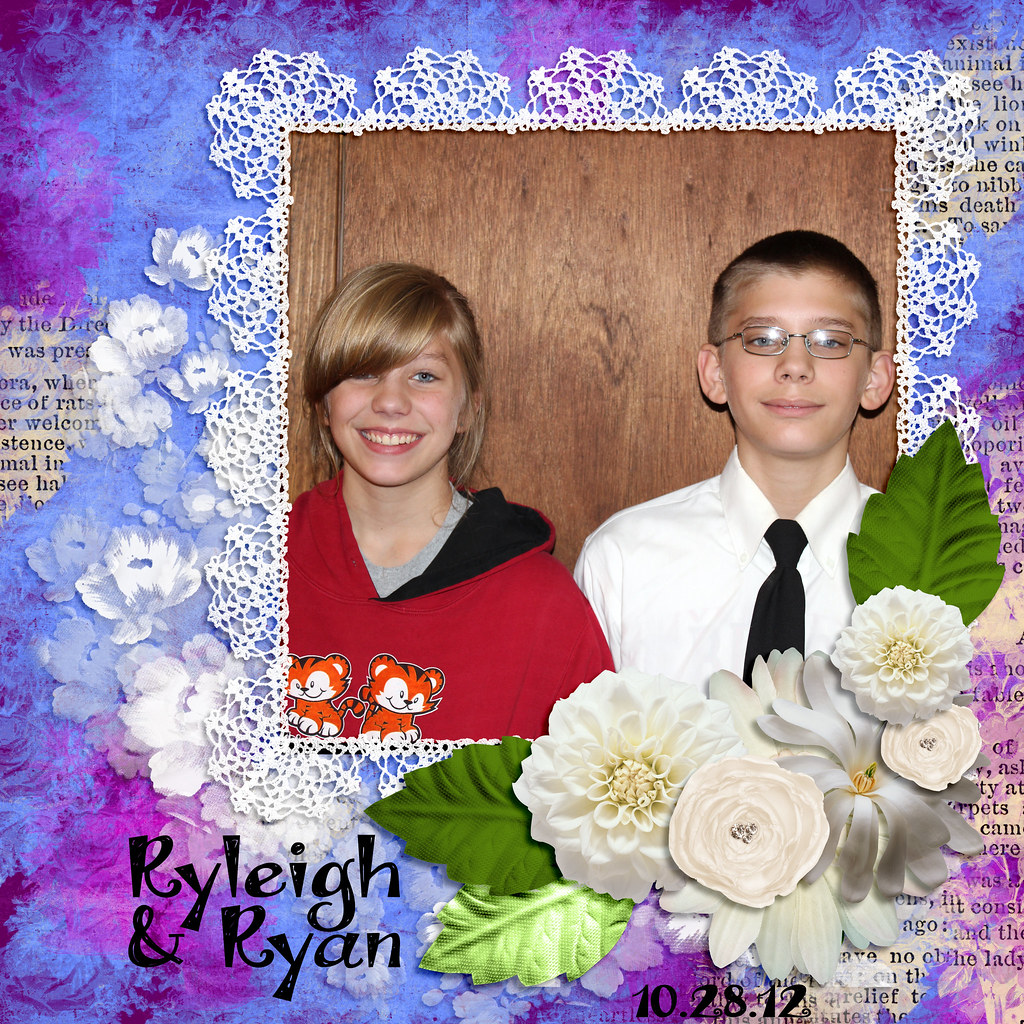The image showcases a meticulously scrapbooked photograph of two young Caucasian children, centered on a batik-styled background that transitions between shades of blue and purple. The background features hints of newspaper snippets and indecipherable printed lines, adorned with lace and floral accents. The photograph itself, framed by delicate lace, reveals a blonde girl with light eyes and a radiant smile, dressed in a red top with critters on it over a gray shirt. Standing to her right is a boy with closely cropped hair, sporting square glasses and a white shirt paired with a black tie. Surrounding them are intricate details: anime-style animal characters on the left, and flowers with green leaves on the right. At the bottom of the page, in an elegant black font, are the names "Riley and Ryan," alongside the date "10-28-12." The overall composition, rich with hues of blue, purple, gray, white, black, pink, red, orange, and brown, creates a multi-textured, vibrant collage, capturing a nostalgic moment with artistic finesse.